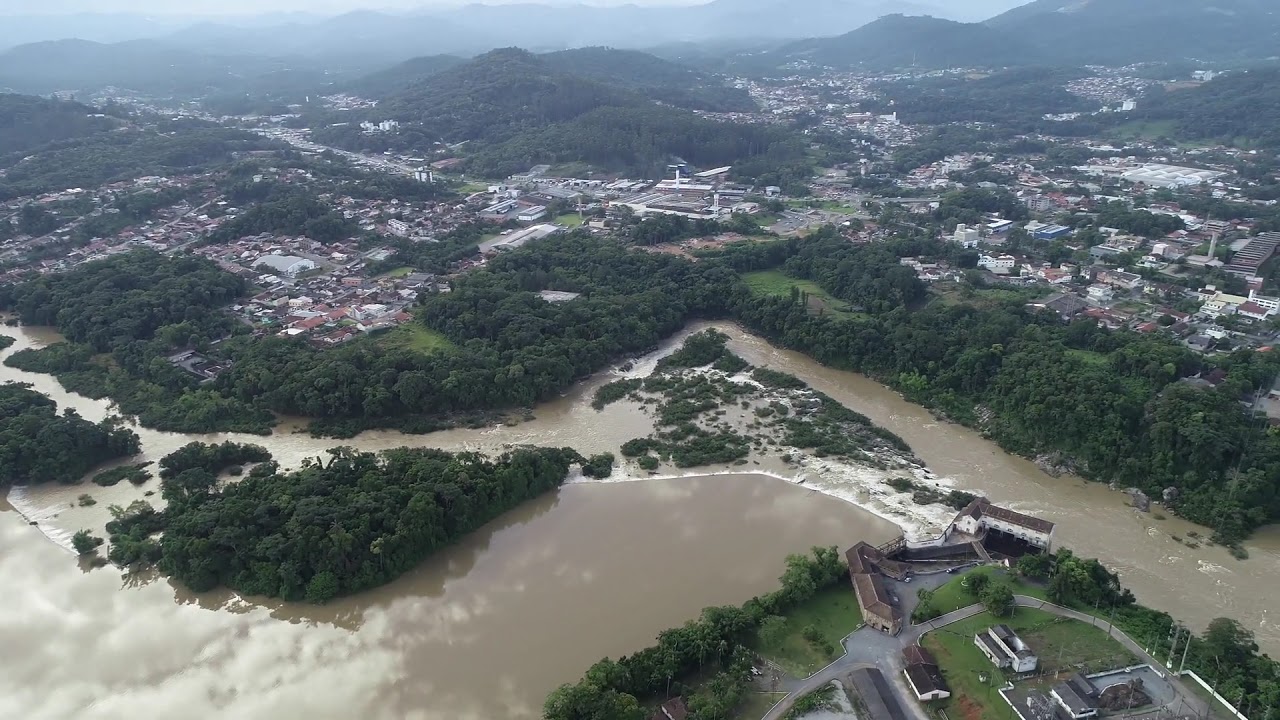This image is a detailed aerial view, possibly taken from a helicopter, airplane, or drone, showcasing a vibrant wetland area with a dark brown river flowing through the scene. The river meanders centrally from left to right, forming a triangular delta in the middle. Surrounding the river is a dense border of heavy trees, framing the scene with lush green foliage. 

In the foreground, the river’s light brown, muddy waters have areas of rough, white water, indicating possible flood conditions. Near the bottom right, there's an island area with a few commercial buildings. On either side of the river, sections of housing are visible, with clusters of homes interspersed with tree cover, stretching into neighborhoods and roads.

Further back, low-lying hills give way to a mist-covered mountain range that dominates the distant background, adding a dramatic element to the landscape. The absence of text or people in the image allows the natural and built environment to provide the primary focal points. The image captures the interplay between the natural wetland and the built environment, set under a hazy, mountainous backdrop, all viewed through the lens of drone photographic realism.